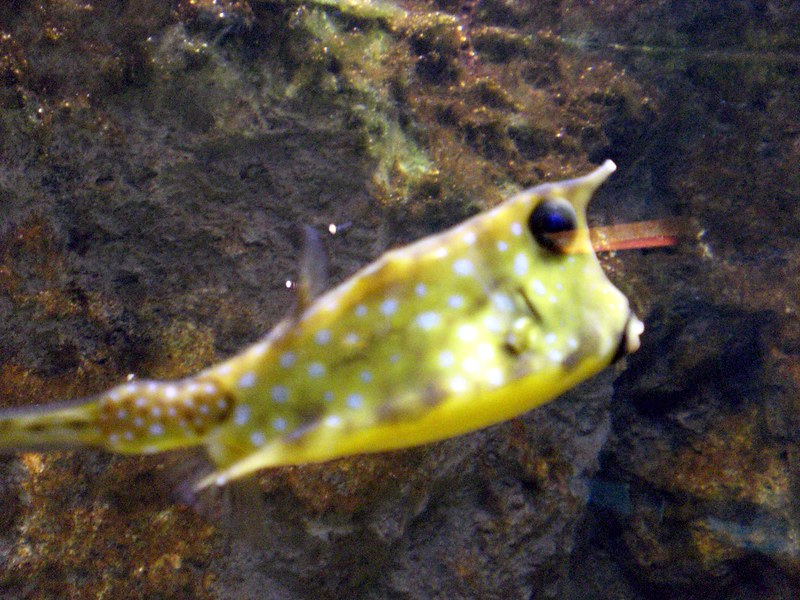The image showcases a distinctive fish within a fish tank set against a backdrop of coral rocks and seaweed-laden stones. The fish, centrally positioned and slightly blurry, boasts a bright yellow body adorned with brown and white dots. Its form is both unique and almost abstract, featuring a slender, pointed nose, and bulging eyes with a mixture of black, brown, and blue colors. The fish’s body curves softly, while the top remains relatively straight. It is punctuated by delicate, slender fins along its sides, a small fin near its tail, and an additional fin atop its head. Light plays off the fish's almost translucent skin, casting subtle highlights. The background is rich with gray rocks, green moss, and muted coral hues, adding depth and contrast to the vibrant subject in the foreground.